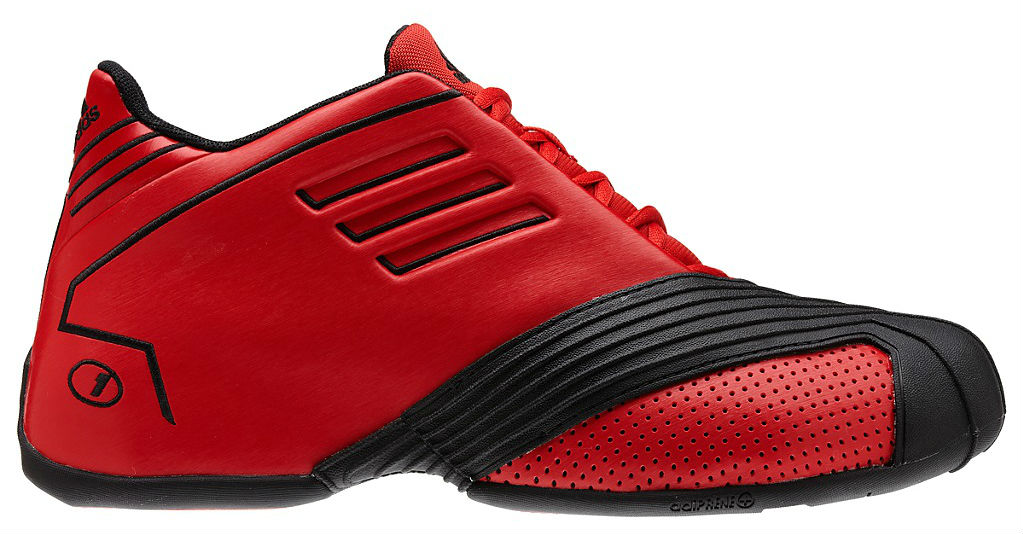This detailed photograph features a predominantly red sports sneaker designed for the right foot, likely from 2024, possibly by Adidas. The shoe is set against an invisible rectangle on a white background, creating a seamless look. The design integrates various textures and patterns, emphasizing both functionality and aesthetics.

The toe of the sneaker is covered by a distinct black piece that wraps around and extends diagonally towards the center and then curves down over the toe area, embellished with black and gray textured stripes. Underneath this black piece, there is a section of red material, likely featuring rows of small, cross-aligned air holes arranged in a square pattern.

The upper part of the shoe, including the tongue, is red, and it is equipped with red shoelaces. Below the tongue, on the lower left, there are three carved-in rectangles aligned horizontally but also appearing diagonal. Adjacent to these, a black stripe extends in a complex path – diagonally down to the left, then vertically downward, and continuing diagonally downward to the right.

Towards the heel of the shoe, a rounded black circle containing a number "1" is noticeable. The summit of the shoe's upper left side features three black diagonal stripes, sloping downwards from right to left. The sole of the sneaker is black, completing the sleek, modern design intended for sports performance.

Overall, the sneaker boasts a triangular shape with the longest side outlining the front and bottom, making it a standout piece potentially aimed at the high-performance sports market.